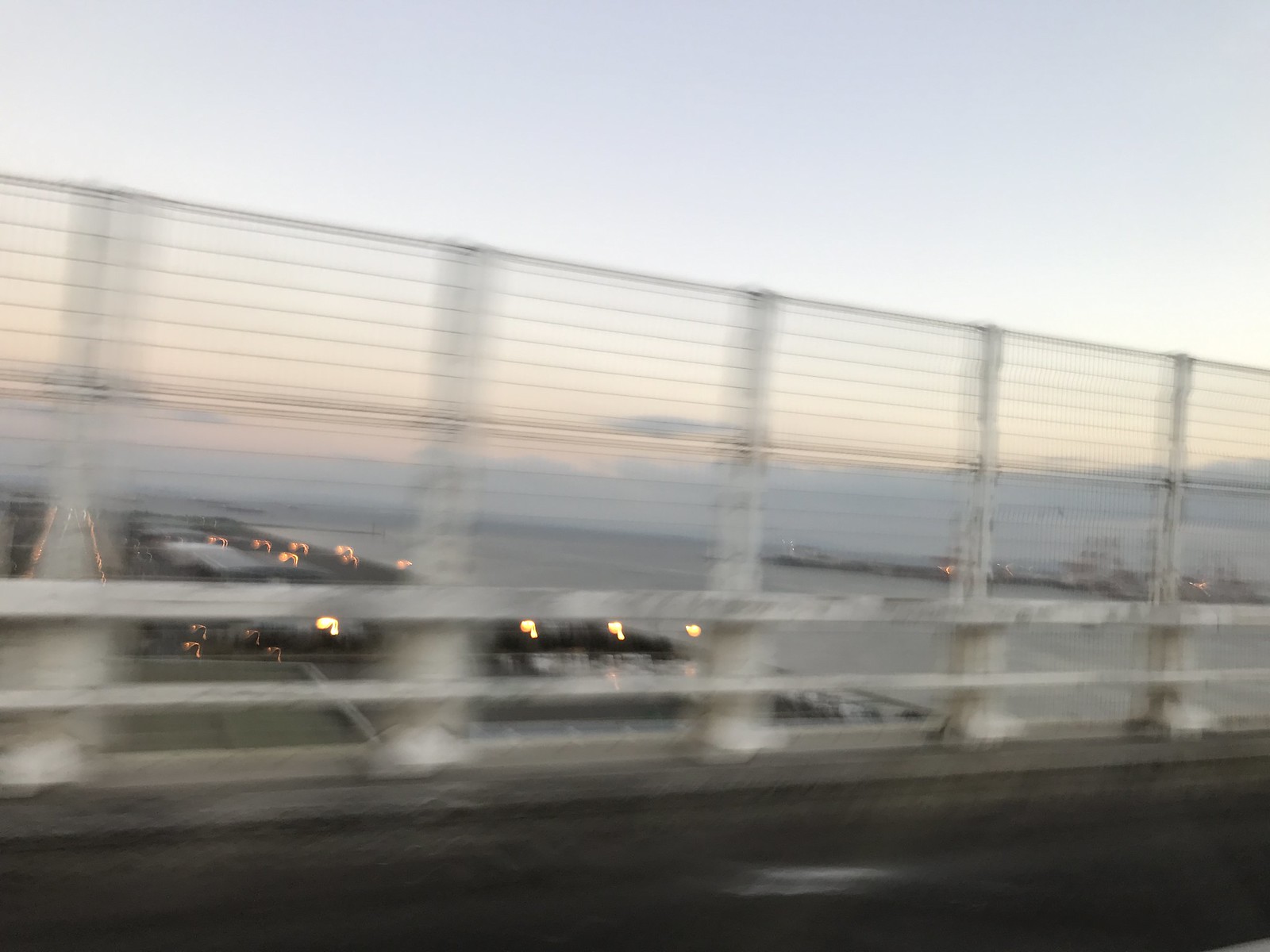A blurry photograph captured from a moving vehicle crossing a bridge. The rectangular image primarily exhibits a vivid sky, transitioning from light blue at the top to warm hues of yellow and orange near the horizon. Dark gray clouds scatter across the sky, dominating the horizon line. In the foreground, the gray asphalt road is bordered by a short concrete curb. Above the curb, a white painted metal railing with a wire mesh fence adds definition. Below this fence, hints of multiple buildings can be seen, occupying a lower level beneath the bridge. The overall composition creates a sense of motion and depth, framed by contrasting elements of urban infrastructure and a dynamic sky.